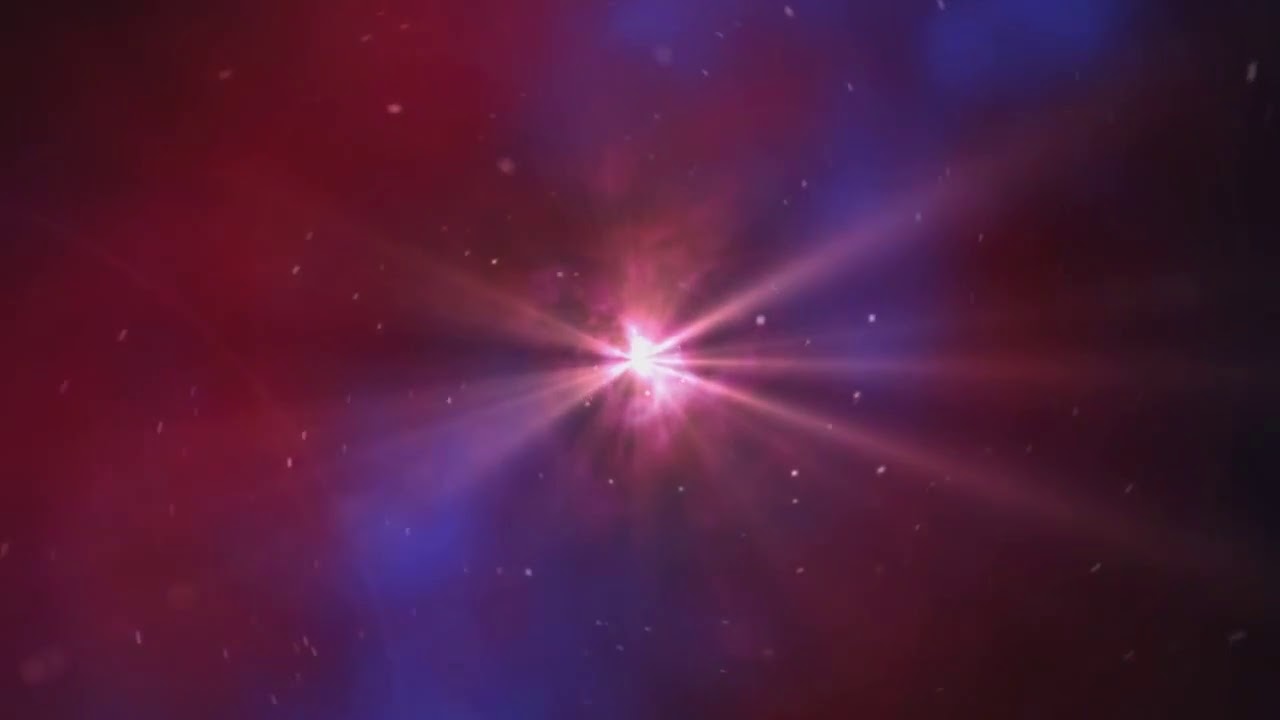In this detailed, computer-generated image, we observe a mesmerizing depiction of space, featuring a vibrant and energetic galaxy or constellation-like scene. The centerpiece of the rectangular frame is a blinding burst of white light, reminiscent of a galaxy on the brink of explosion or a black hole emitting radiant beams. Its brilliance stretches left and right, casting streaks of light across the image.

Surrounding this central burst are swirling patterns of light and colors that include vivid blues, soft reds, and delicate pinks, giving off a tie-dye appearance. Numerous white dots, representing stars or stardust, are scattered throughout the background, some areas appearing slightly blurred to add depth. These dots seem to follow a circular or cylindrical motion, suggesting the immense gravitational pull of the central phenomenon.

On the outer edges, particularly towards the right, the colors gradually fade into a black expanse, emphasizing the contrast and vastness of space. The image, with its rich palette and intricate details, exudes a strikingly sci-fi atmosphere, highlighting the enigmatic and captivating nature of the cosmos.